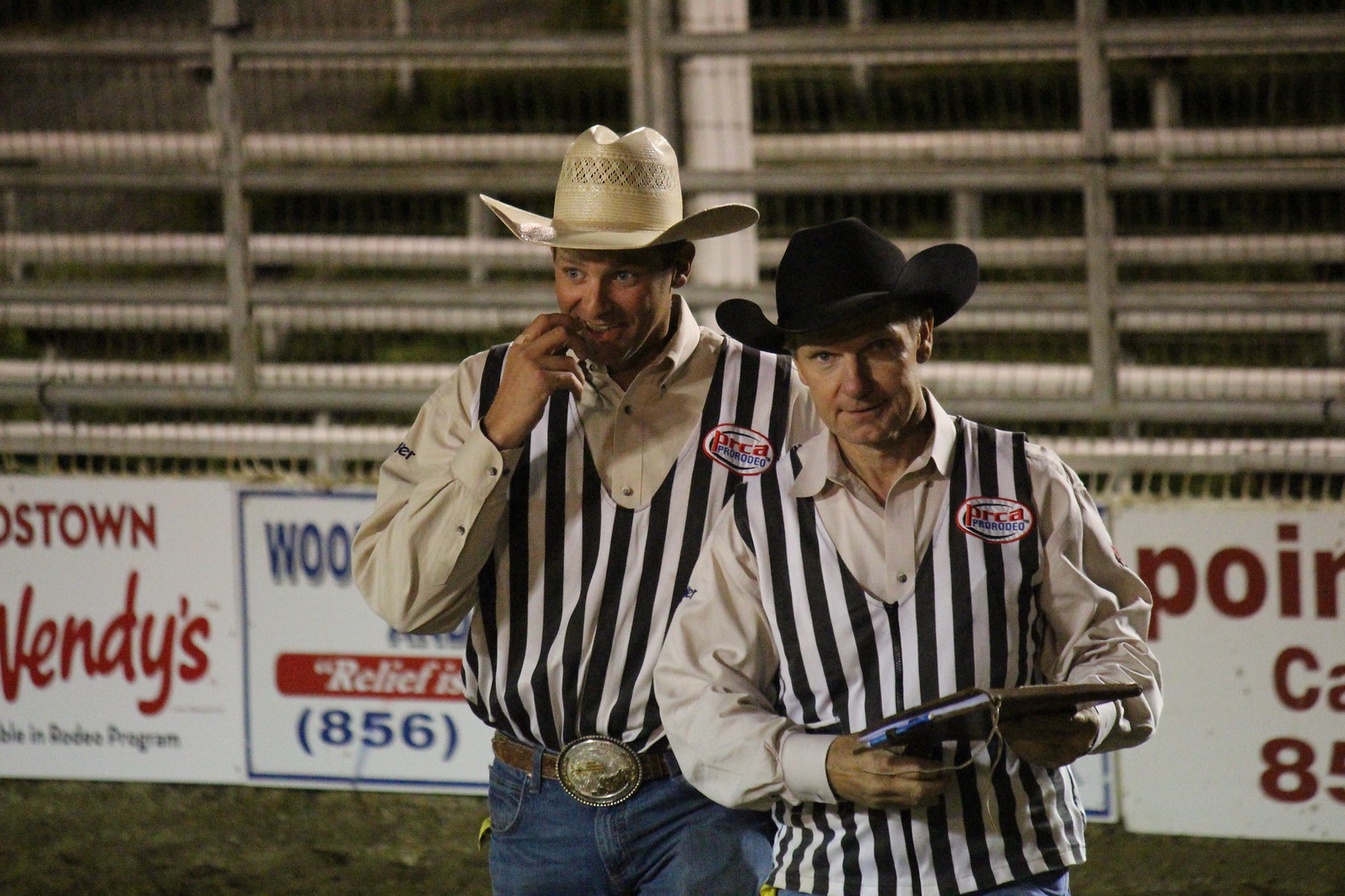This is a detailed photograph featuring two Caucasian men, likely in a rodeo setting at nighttime. The background reveals a silver metal fencing typical of a rodeo arena, with visible advertisements below it, including one with the Wendy's logo. Both men are front and center, adorned in black and white vertically-striped vests with the logo "PRCA" on them. They are dressed in white shirts under the vests. The taller man on the left sports a tan or off-white cowboy hat and notable attire, including a large silver belt buckle and denim blue jeans. His right hand is touching the side of his face as he gazes to the left. The man on the right is slightly shorter, dons a black cowboy hat, and holds what appears to be a tablet in a brown leather case. A pin or accessory is noticeable on his vest. The ground they stand on seems to be dirt or straw, fitting the rodeo environment. Behind them, no crowd is visible, adding to the sense of an empty or after-hours arena. Both men stand looking in different directions, immersed in the open, spacious rodeo field.